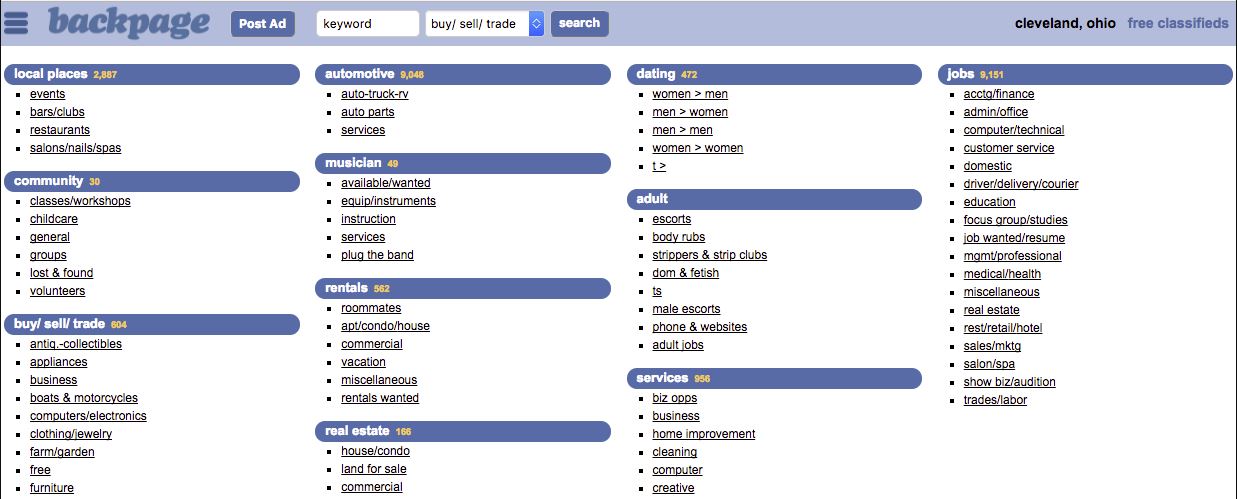**Detailed Description of Backpage Screenshot:**

The screenshot captures the main interface of the Backpage website. The top navigation bar is colored in a light blue hue. In the top-left corner, there is a menu icon resembling three stacked horizontal lines, commonly known as a "hamburger" menu. Adjacent to this icon, the title "Backpage" is prominently displayed.

Beneath the title bar, there is a button for posting an ad. The search functionality is positioned centrally, featuring a white text box labeled "keyword" and another white box with the inscription "buy/sell/trade" in black font. These boxes are accompanied by a search button.

On the far right of the top bar, the text "Cleveland Ohio free classified" is visible, indicating the specific local area the page pertains to.

The content is categorized meticulously:
1. **Local Places and Events:**
   - Bars/Clubs
   - Restaurants
   - Salons
   - Nails
   - Spas

2. **Community:**
   - Classes or Workshops
   - Child Care
   - General Groups
   - Lost and Found
   - Volunteers

3. **Buy/Sell/Trade:**
   - Antique Collectibles
   - Appliances
   - Business
   - Boats and Motorcycles
   - Computers
   - Electronics
   - Clothing
   - Jewelry
   - Farm and Garden
   - Free Items
   - Furniture

4. **Automotive:**
   - Auto/Truck/RV
   - Auto Parts
   - Services

5. **Musician:**
   - Available/Wanted
   - Equipment
   - Instruction
   - Services
   - Plug the Band

6. **Rentals:**
   - Roommates
   - Apartment/Condo/House
   - Commercial
   - Vacation
   - Miscellaneous
   - Rentals Wanted

7. **Real Estate:**

8. **Dating**

9. **Adult Services**

10. **Jobs**

The layout offers a comprehensive assortment of categories, thus providing users with a streamlined experience to locate specific sections relevant to their needs.